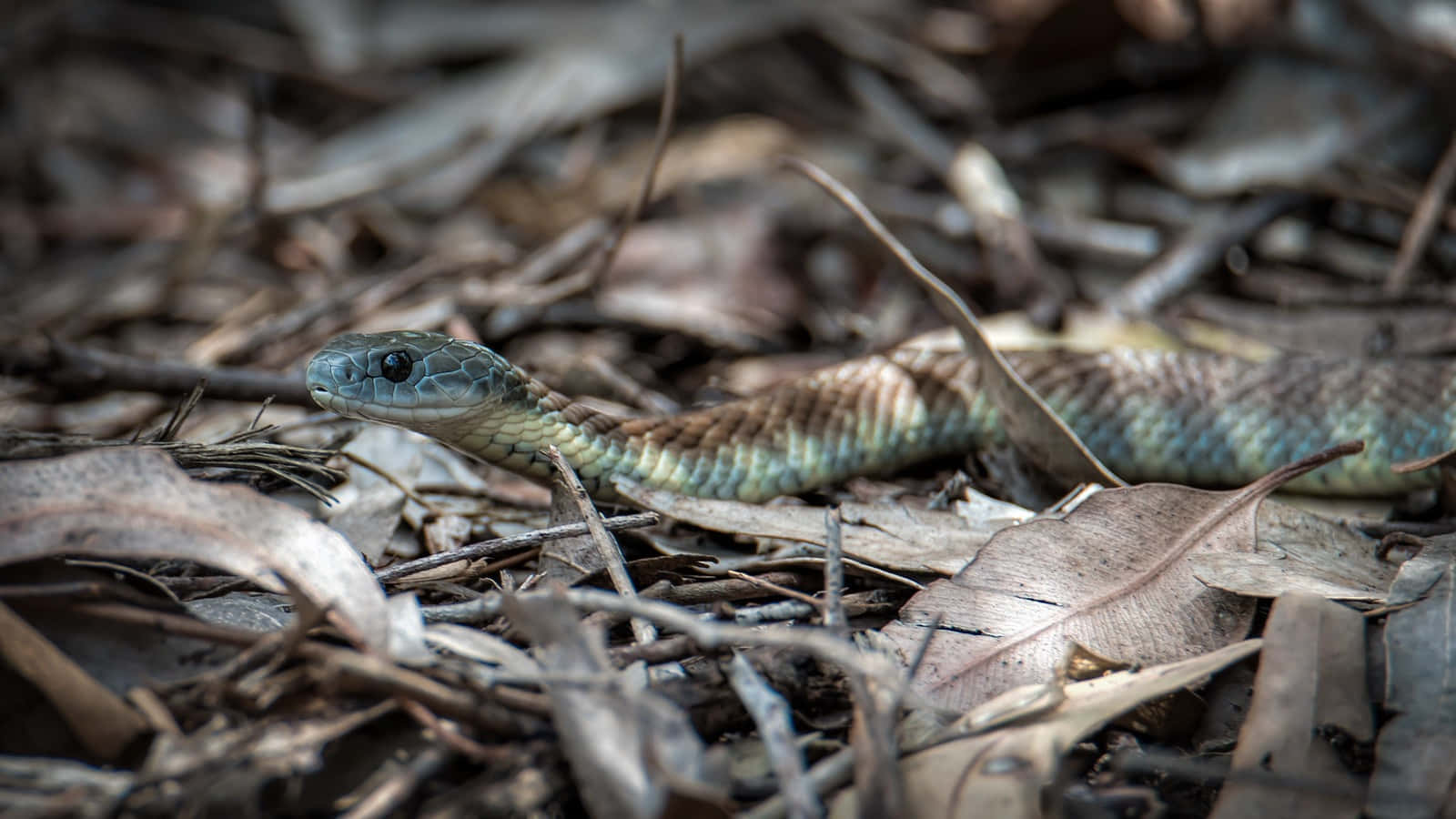This detailed close-up image captures the front end of a snake slithering through a dry, woodsy area filled with brown, crispy leaves and twigs, suggesting an autumn setting. The snake's head, positioned at the left one-third of the rectangular photograph, is a striking bluish-green with white underneath its mouth and noticeable black eyes. The body extends horizontally, revealing dark green scales near the head transitioning to a creamy white underside and a predominantly brown back with some greenish-blue hues mingled in the lower portions. The background is blurred, emphasizing the snake's scales and lines with clarity, enhancing the texture of its skin. The scene is dappled with a bit of sunshine, adding to the natural, serene ambiance of the image.